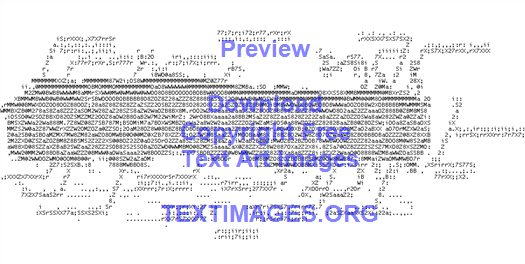The image is an attempt at ASCII art, featuring black characters on a white background. ASCII art typically uses letters, numbers, and symbols to create images, but in this case, the result appears jumbled and unclear. The text forms an indiscernible shape in the center of the page, resembling a bumpy oval with lines and squiggles extending from it, possibly suggesting the legs of a bug or a centipede. However, it's difficult to determine the exact figure. Overlaying this chaotic arrangement is a transparent blue or purple font that reads "Preview, Download, Copyright-Free Text Art Images" and "TextImages.org" at the bottom. The overall impression is one of a poorly defined image made from a myriad of tiny characters, with promotional text emphasizing its availability for download.